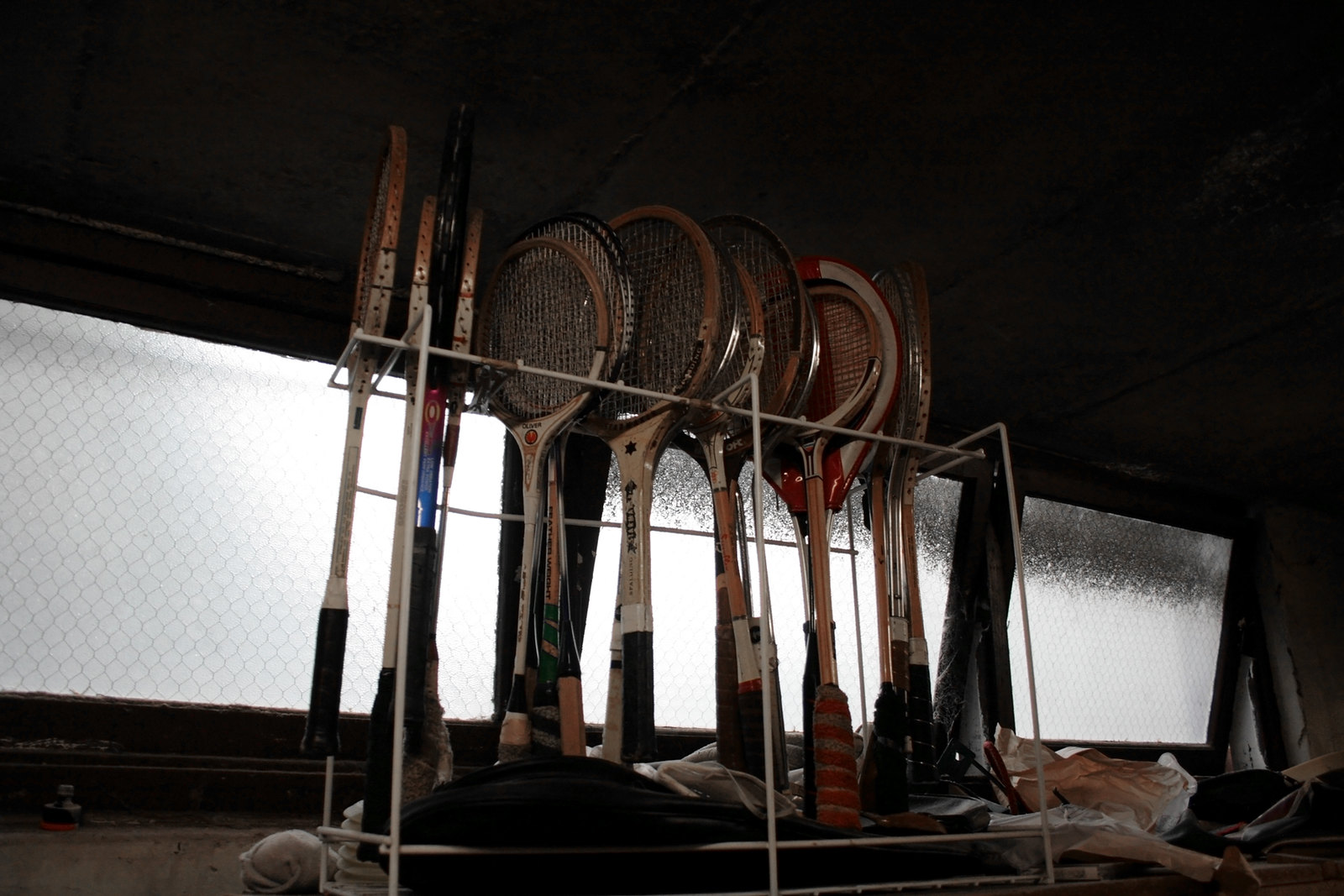This photograph features a rack holding approximately 10 to 12 rackets, with a mix of tennis and badminton rackets. The rackets showcase various designs and conditions: some have the traditional oval shape typical of tennis rackets, while others are more rounded, characteristic of badminton rackets. The handles of these rackets vary in color, including black, red, and blue, with some wood-toned ones visible as well. The rack is positioned in front of a large, fogged-up window reinforced with chicken wire and framed in black trim, suggesting an old, possibly basement-like or storage environment. The window also reveals a gray, overcast outdoor scene. The lighting is dim, creating a dark and somewhat shadowy atmosphere. Below and around the rack, there are piles of cloth or fabric, adding to the sense of clutter and age in this storage space. The image angle seems to be slightly from below, looking up at the rack and the window.